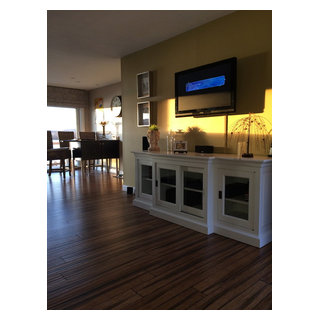The image depicts the interior of a cozy house or apartment living space. On one wall, a flat-screen TV is mounted above a sleek, white hutch featuring glass doors and multiple shelving units. Atop the hutch, various decorative items, including picture frames, a candle, and a small potted plant, add a personal touch to the space. The room is adorned with wooden flooring and the walls are painted in a warm, beige-brown hue. Natural sunlight brightens part of the wall, while the rest of the room remains in soft shadow.

To the left, there is a window that allows additional light to filter in. A dark-colored dining table accompanied by matching chairs is situated near this window. Behind the table and chairs, a large window provides an expansive view, suggesting plenty of natural light during the day. On the wall above the dining area, a clock is also visible. The table seems to be decorated with what looks like a candlestick, although the small size of the image makes finer details challenging to discern.